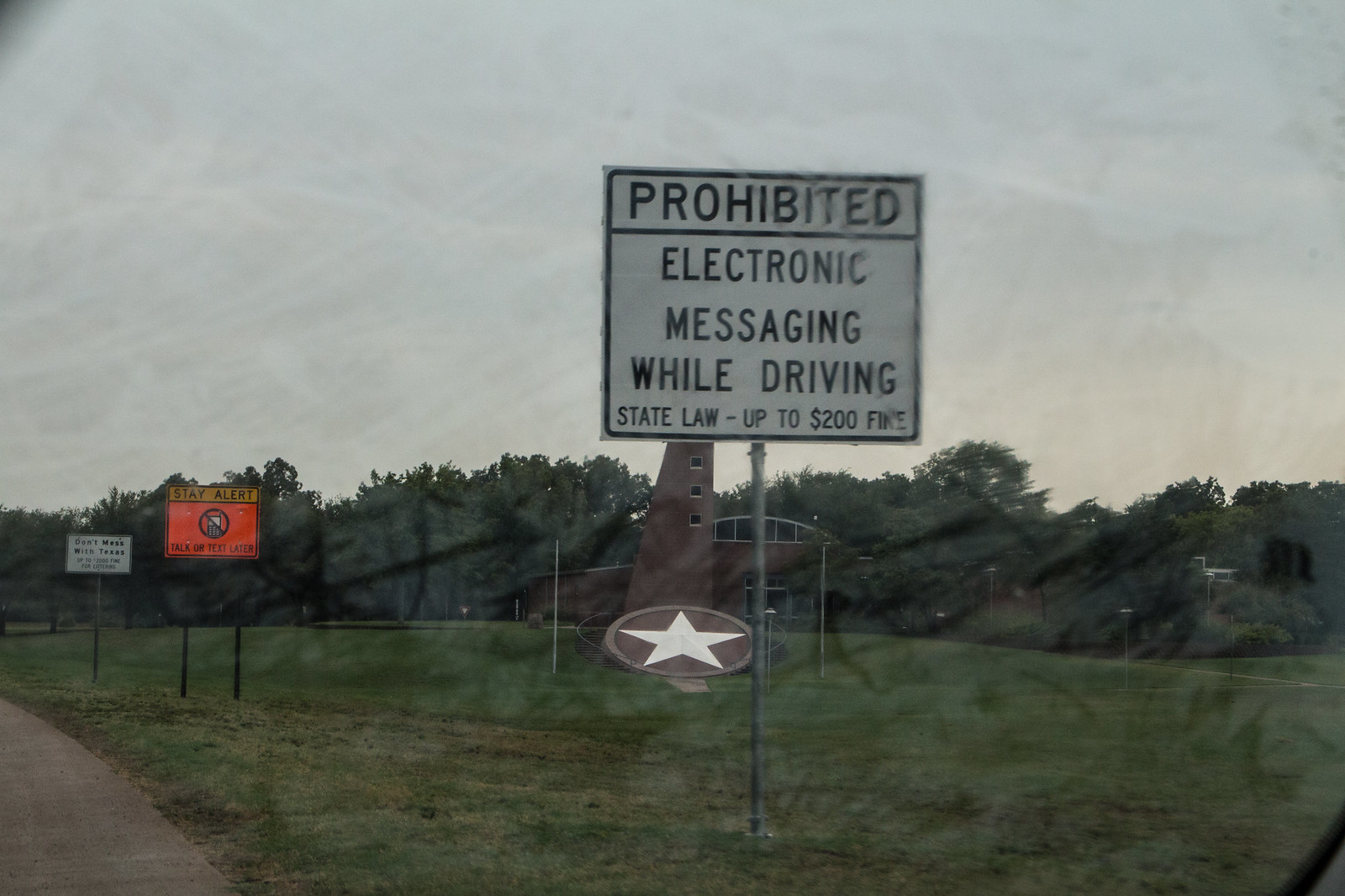This color photo, taken through a smudged car window marked with fingerprints, features a prominent white sign with black lettering in the center. The sign, mounted on a gray pole, reads "Prohibited Electronic Messaging While Driving - State Law - Up to $200 Fine." Beyond this sign, a brick-colored building with an arched roof and upper windows stands tall, partially obscured by the sign. At its base is a large, round emblem with a white star, propped up rather than lying flat, hinting at a possible army base. To the left, a bright orange digital sign supported by black poles displays the words "Stay Alert." Further down the grassy area where the building is situated, additional signs and a row of tall green trees frame the background. The sky is overcast with white and gray clouds, indicating it might be late afternoon or evening.